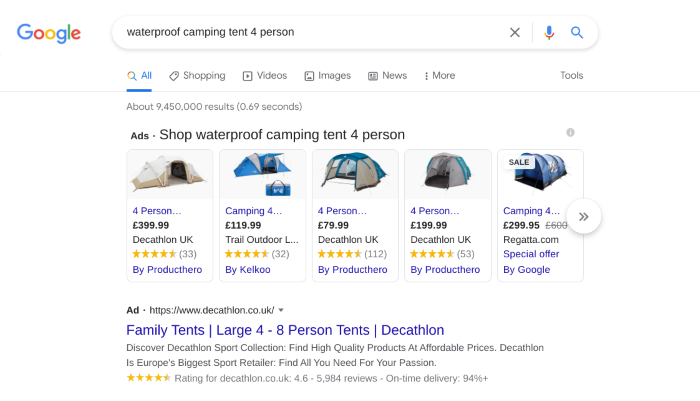This image is a well-detailed screenshot of a Google search result for the query "waterproof camping tent for person." The screenshot displays various elements typical of a Google search results page and offers a clear visual representation of the search interface.

At the very top-left corner, the iconic Google logo is prominently displayed, with its distinct multicolored letters (blue, red, yellow, and green). Centrally positioned at the top, the Google search bar contains the exact search phrase "waterproof camping tent for person." On the far right of the search bar, a small black "X" icon allows users to clear the query, followed by a light gray vertical bar, a blue microphone icon indicating the voice search option, and a blue magnifying glass, which is the search button.

Immediately below the search bar, a navigation menu offers different content types that users can explore. The menu options include "All" (highlighted in blue to indicate the current selection), "Shopping" (accompanied by a small shopping tag icon), "Videos" (with a video clip icon), "Images" (displayed with a photo icon), "News" (with a newspaper icon), and "More" (represented by three vertical dots). To the far right of this menu, "Tools" is available in gray text for further search customization.

Directly below this menu, in light gray text, it is indicated there are approximately 9.45 million results returned in 0.69 seconds. The main focus of the page is a large advertisement in the center, urging users to "Shop waterproof camping tent for person," showcasing five different tents of various designs and colors from multiple websites.

At the bottom of the image, the first search result is another advertisement from the website decathlon.co.uk. It invites users to explore family tents, specifically large four to eight-person tents, from Decathlon. Below the link, there's a brief description of the site, its ratings, and some customer reviews, providing additional details to guide potential buyers.